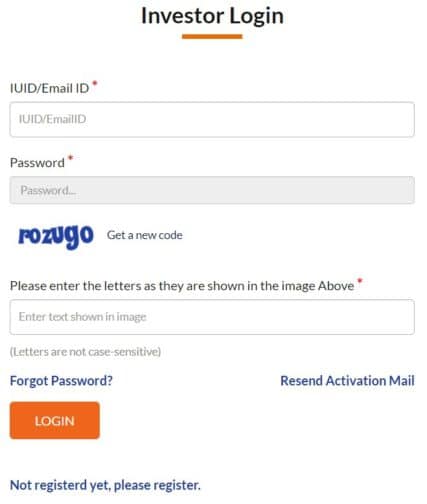This image depicts an investor login opt-in form designed with a clean and modern interface. At the top of the form, the heading "Investor Login" is prominently displayed with a sophisticated gold underline, adding a touch of elegance. Below this heading, users are prompted to enter their email address and password into dedicated input fields. The form includes a CAPTCHA challenge to verify human interaction, ensuring security and preventing automated access.

Further down, users are instructed to enter a code, which is written in blue font. It is noted that the letters in the code are not case-sensitive, simplifying the input process. For users who may have forgotten their password, there is a "Forgot Password" link also in blue text, allowing them to initiate the password recovery process.

At the bottom of the form, an orange "Login" button is prominently displayed for users to submit their login credentials. Additionally, for new users who have not yet registered, there is a "Not Registered" link, which provides options to create a new account. This comprehensive and user-friendly form ensures a seamless experience for investors looking to access their accounts.